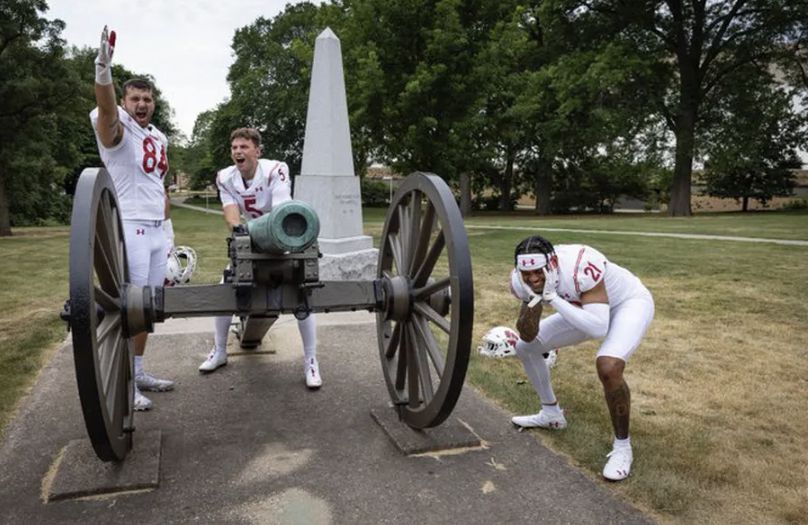In this detailed and descriptive scene, three high school football players are posing around a vintage, green war cannon displayed on a grassy lawn. The cannon, which has very large wheels, is set against a backdrop featuring a white, slender, pyramid-like memorial statue bearing some inscriptions. The players, dressed in white jerseys with red lettering, complete their uniforms with various lengths of white socks, cleats, gloves, and helmets placed on the ground. 

The image captures them in a playful yet dynamic moment as one player stands to the right, seemingly plugging his ears to mimic the sound of a cannon blast, while another energetically shouts "charge," and the third pretends to fire the cannon. They are surrounded by a lush landscape with trees lining a paved path that runs alongside the grassy area, and patches of a vast green field under a clear, daytime sky. The scene suggests a mix of historical reverence and youthful exuberance, potentially situated at a famous college or memorial site.